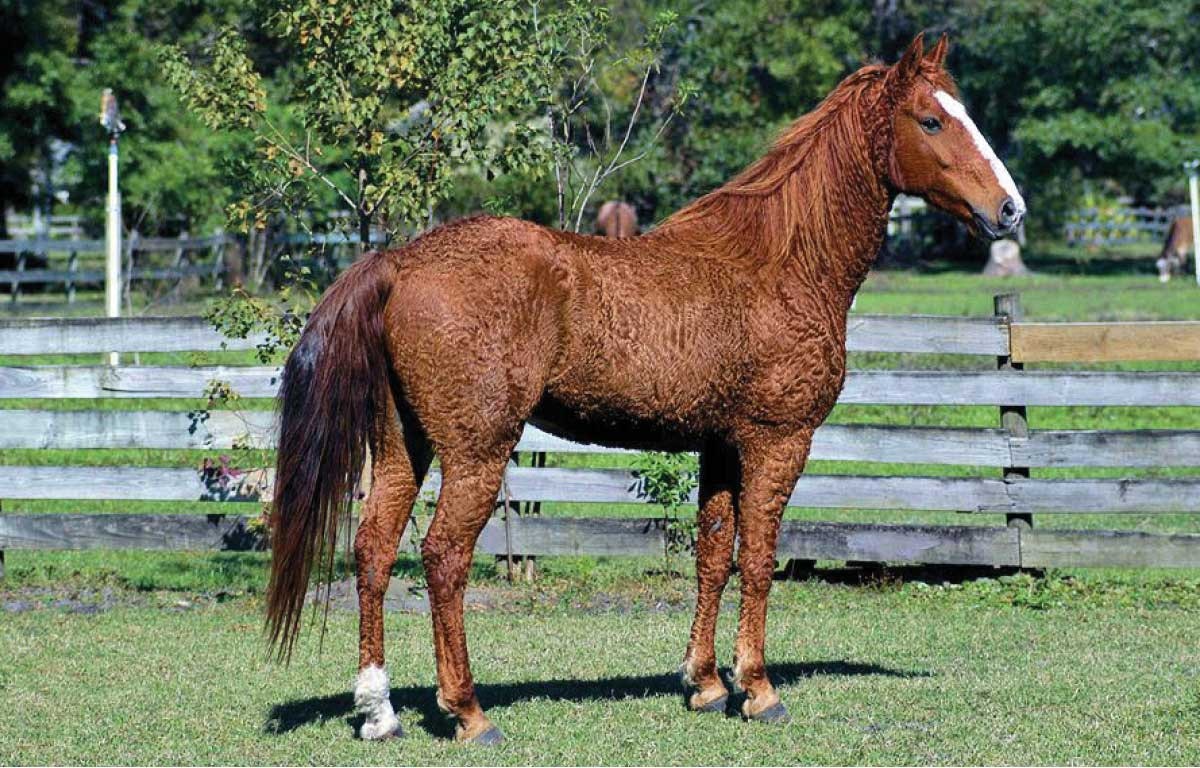A rusty brown horse with a wavy, textured coat stands on lush green grass, facing right, in a charming outdoor paddock. The horse's dark chestnut tail is visible, along with a distinguishing white strip running down its face and a single white back hoof. The scene is framed by an old, gray-toned wooden fence with five rails, set against a backdrop of dense trees and shrubbery, suggesting a serene farm environment. A hint of another animal, possibly a cow, can be seen in the upper right corner. The horse's shadow indicates it's a bright, sunny day. Its mane matches the horse's body color, and one of its dark eyes and nose are clearly visible as it gazes calmly forward.